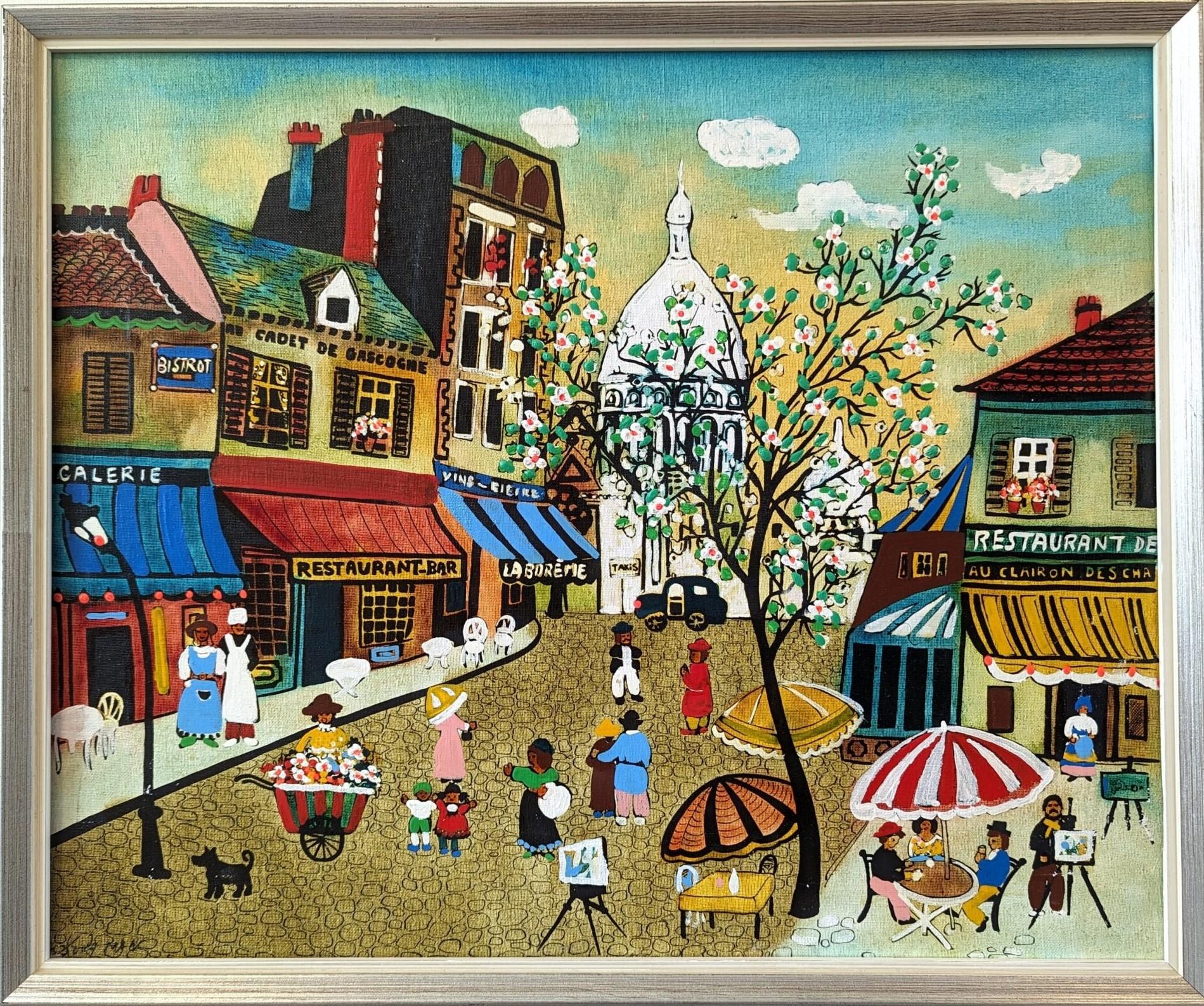The painting is an artistic rendering of a vibrant and bustling street in a small town, filled with vivid colors and intricate details. The foreground features a tree with black bark, adorned with white flowers that have yellow and pink centers, standing adjacent to a unique, bent streetlamp under which a small dog sits. The cobblestone street is alive with activity: people are walking, a flower-seller stands mid-street, surrounded by two children and a woman with an outstretched arm, and another woman in a pink dress holding an umbrella strolls with her back to the viewer. 

To the right, there's a restaurant with brown roof tiles and a red chimney, flanked by potted plants and displaying a mix of open and closed windows. Its outdoor seating area includes a red-and-white umbrella, where diners gather around a table, and a nearby artist in a black shirt and brown pants captures the scene on canvas. The left side of the street is lined with colorful storefronts and eateries, such as one with a blue sign and awnings, and another with green trim, a red roof, and a yellow awning, labeled "Restaurant Bar" and "Calary" or "Colerie." In one of these outdoor spaces, people sit at a table under a red-and-white umbrella.

A small government building with a steeple and a black car parked in front is visible in the distance, partially obscured by the blooming tree. The sky transitions from cyan to yellow and orange, indicating the time of day, and a taxi cab can be seen in the far background, contributing to the lively atmosphere. The scene is anchored by the underlying suggestion of a French locale, with signs like "Cadet de Gascogne," evoking a sense of place reminiscent of France or a French-speaking area.